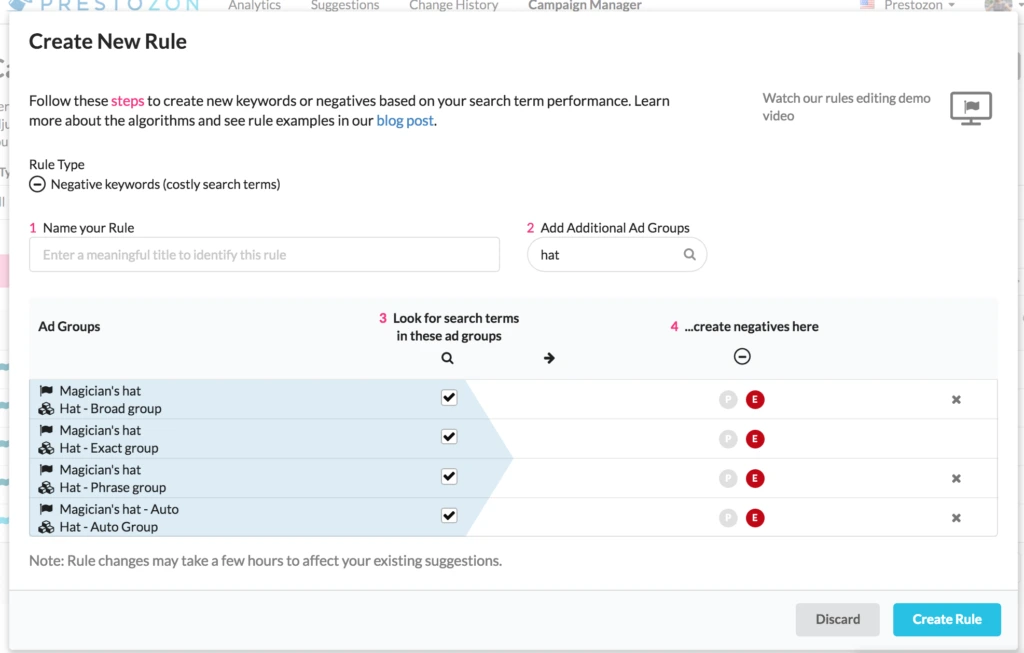The screenshot depicts a web page belonging to a company with a blue logo that appears to say "PRESTOZON" in the top left corner, although the upper part of the letters is cut off. This page is focused on keyword and negative keyword management, featuring several tabs in the toolbar that include "Analytics," "Suggestions," "Change History," and "Campaign Manager." There is also a location icon located at the top right side of the screen.

Overlaying the main background is a large text box with a white background. At the top left of the pop-up box, it says "Create New Rule" in bold text, followed by a set of instructions on how to create new keywords or negatives based on search term preferences. Additional resources are offered, such as a blog post about algorithms and rule examples, as well as a "Watch Our Rules Editing Demo Video" option accompanied by an icon.

The content is organized into steps, starting with "Rule Type." Step number one is "Name Your Rule," and step number two is "Add Additional Ad Groups." Below these steps is a chart titled "Ad Groups" located at the upper left of the chart. Step number three is "Look for Search Terms in These Ad Groups," where a list including "Magician's Hat" and "Hat-Broad Group" is visible, each with check marks indicating selected ad groups. Step number four is "Create Negatives Here," which contains another column for creating negative keywords, with an 'X' icon at the end of each text box for discarding entries.

At the bottom right corner of the image, there is a blue "Create Rule" button, which allows the user to finalize the creation of new rules based on the selected criteria.